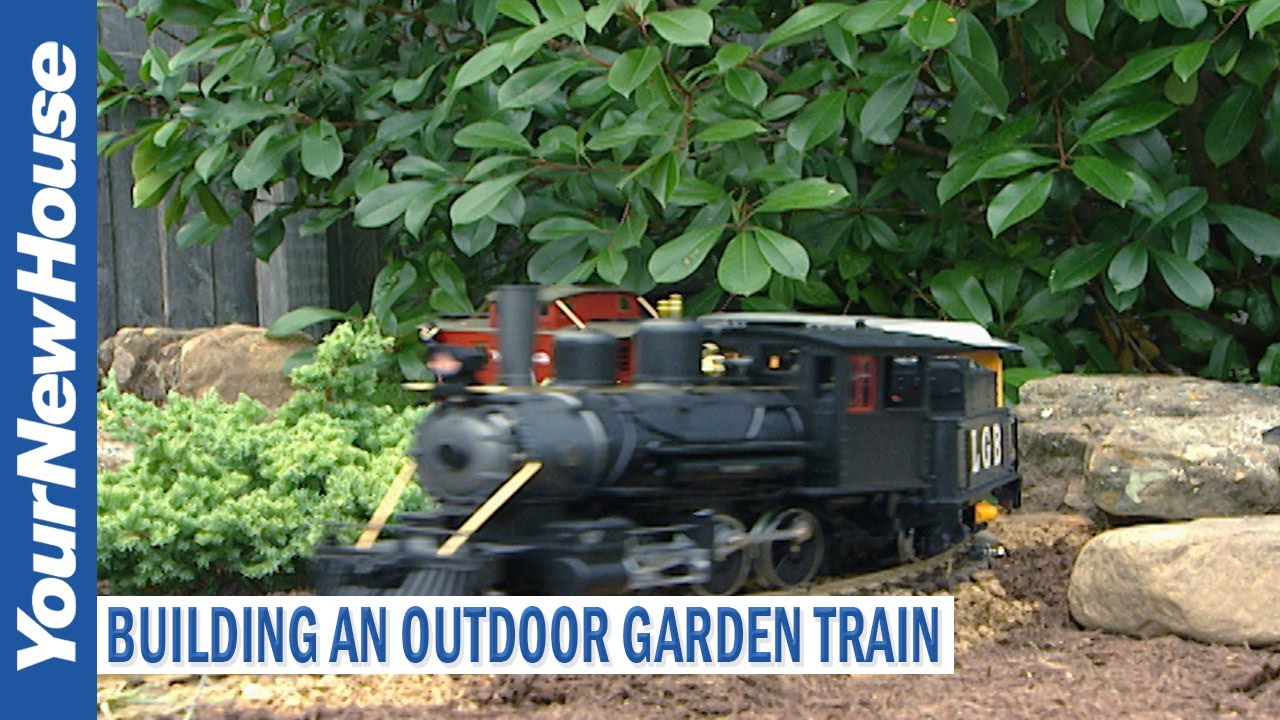This landscape-oriented color photograph showcases a detailed scene of a toy train set in an outdoor garden environment on a sunny day. The focal point is the small train set, reminiscent of a collector's creation, positioned on tracks that weave through an artfully landscaped area. 

The train itself features a large black engine car at the front, followed by several cars including a yellow one, and culminates with a red caboose partially visible as it curves back to the left. To the right, a cream and beige rock stack sits atop brown dirt, providing a naturalistic touch to the setup. In the background, a mix of green plants and dense green shrubbery adds to the garden's lush appearance.

On the left side of the image, a wood plank fence runs parallel to the tracks, bordered by rocks and green foliage. Notable graphic design elements include a vertical blue stripe with white text reading "Your New House" on the left-hand side, and a horizontal white rectangle with dark blue text stating "Building an Outdoor Garden Train" at the bottom left. This blending of photographic realism and graphic elements creates a visually engaging and detailed representation of the garden train setup.